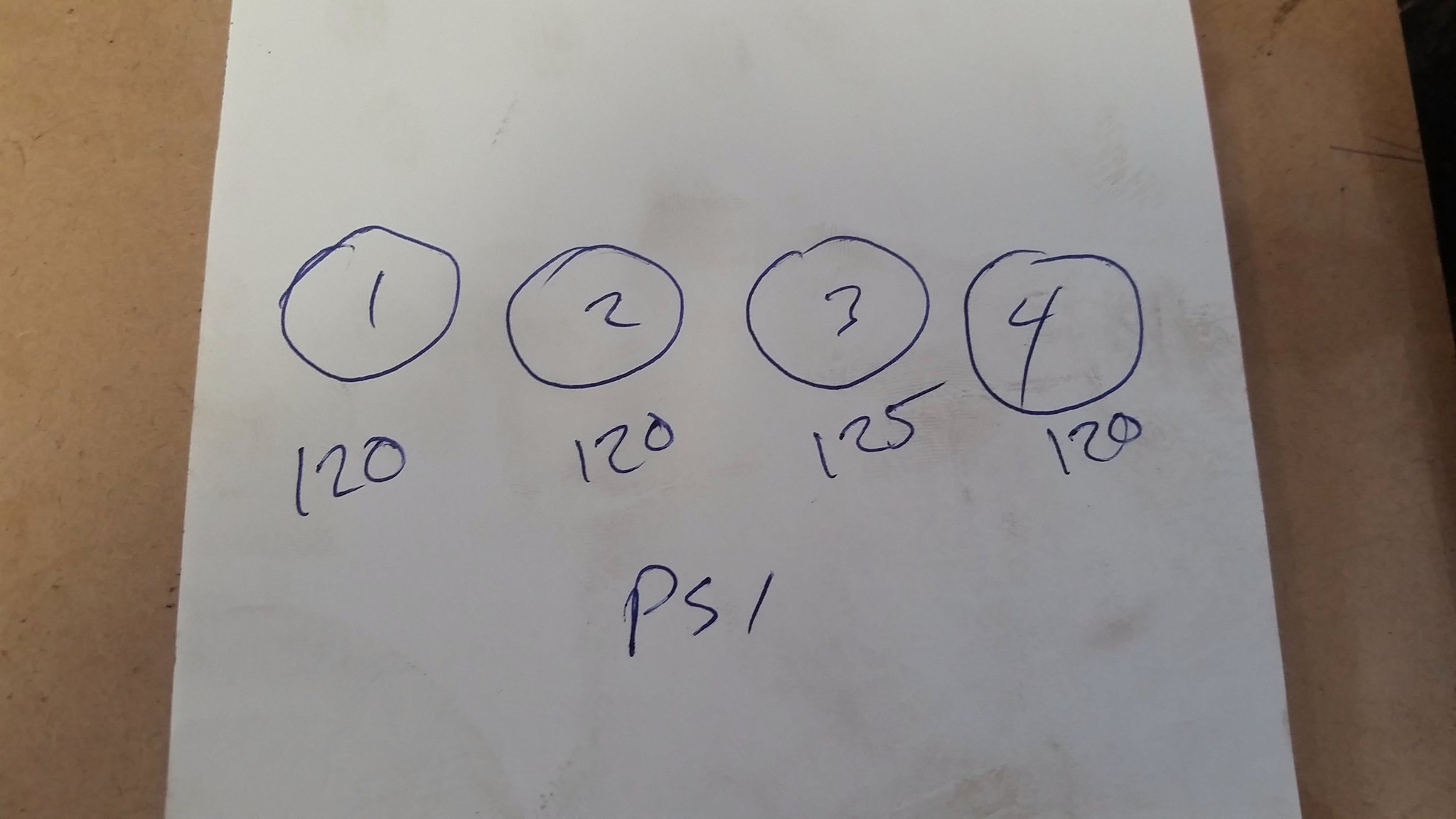A piece of white paper rests on a slightly worn peachy-gray laminate surface, characterized by various scratches and small, intrinsic speckles from its age. The paper features hastily written numbers, one through four, in blue ink, each neatly aligned in a row and enclosed in individual circles. The circles start and end at the top. Beneath each circled number is an additional figure: 120 under both one and two, 125 under three, and 120 under four. Centered below the numbers two and three, the capital letters "PSI" are prominently displayed. The paper is marred by numerous grayish-brown smudges, suggesting it was handled with dirty hands or came into contact with a soiled surface.